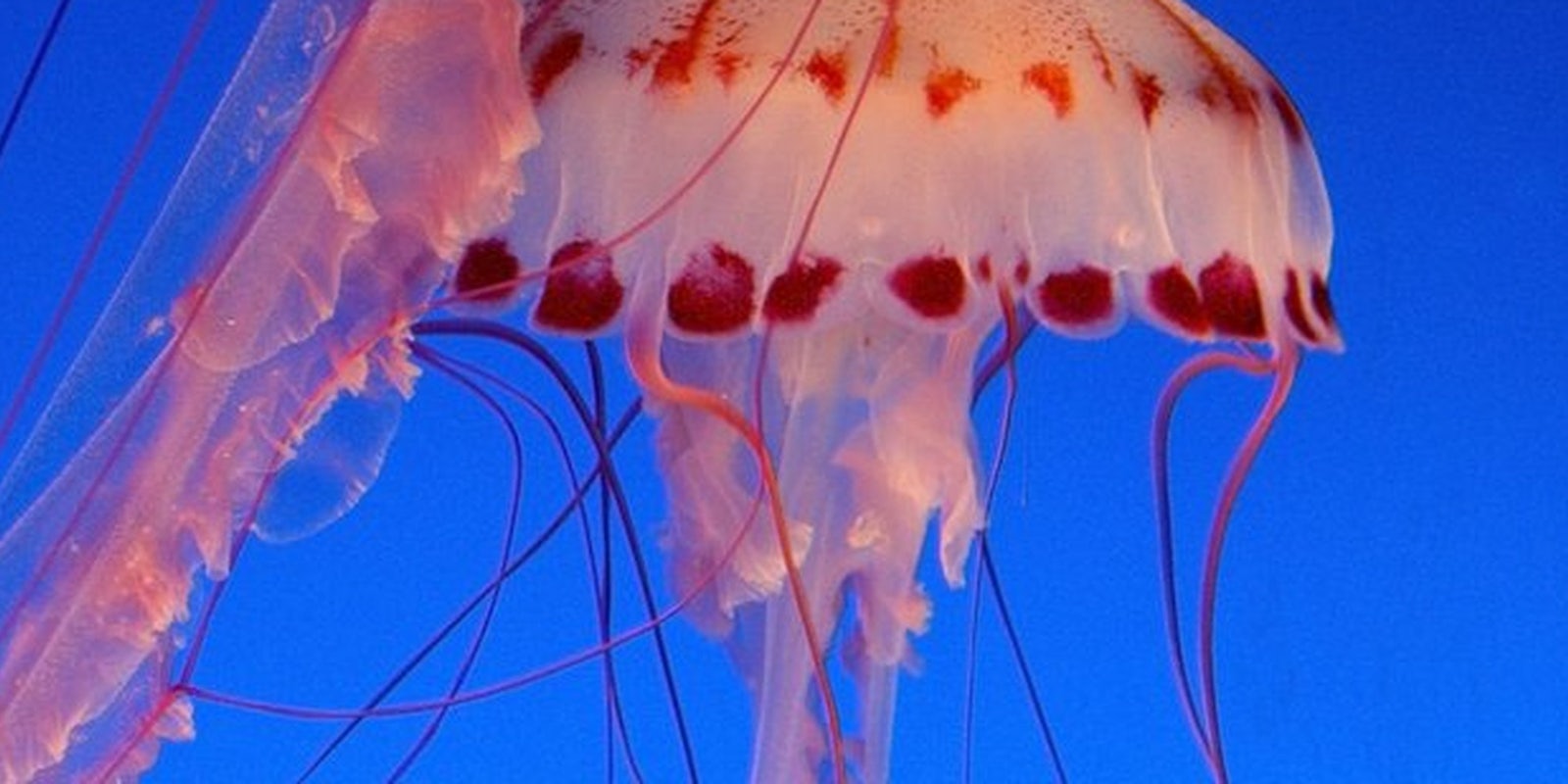This detailed photograph showcases a jellyfish positioned prominently in the center of the frame, against a gradient blue ocean backdrop that transitions from slightly dark to lighter hues, emphasizing the clarity and purity of the water. The jellyfish, predominantly light pink, exhibits an array of colorful nuances and intricate structures. Its somewhat truncated head features a delicate play of darker red markings on its frilly lower edges, adorned with several dark red spots. The body appears translucent pink, with pinkish, reddish, and even some blackish tendrils gracefully trailing below. Notably, its primary stems and stringy structures display variations from milky-clear and pink to deeper reddish hues. Floating upright, the jellyfish’s numerous tentacles, at least ten visible ones, extend elegantly, creating a mesmerizing visual in this real-life oceanic capture.